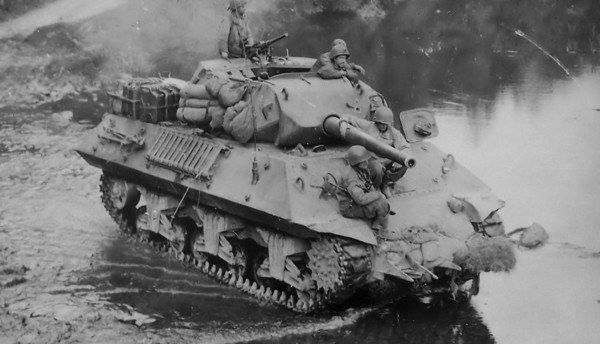In this detailed black-and-white photograph, we see a military tank navigating over a flat, wet surface towards a body of water, indicated by the reflections and ripples on the ground. Positioned centrally in the image, the tank is moving in the direction of a dam visible on the right side. The tank is laden with various accessories, including ladders, blankets, and what appear to be gas tanks and other cargo.

There are multiple soldiers spread across the tank. Two soldiers are seated at the front, one situated beneath the barrel and the other near what looks like a missile launch area. Both are wearing helmets. Another soldier, partially visible, is emerging from the top hatch of the tank, with only his shoulders, arms, and head in view. On top of the tank at the rear, another soldier stands behind a shield, manning a rifle and facing the same direction as the tank. In the background, faint smoke can be seen, adding to the wartime atmosphere of the scene.